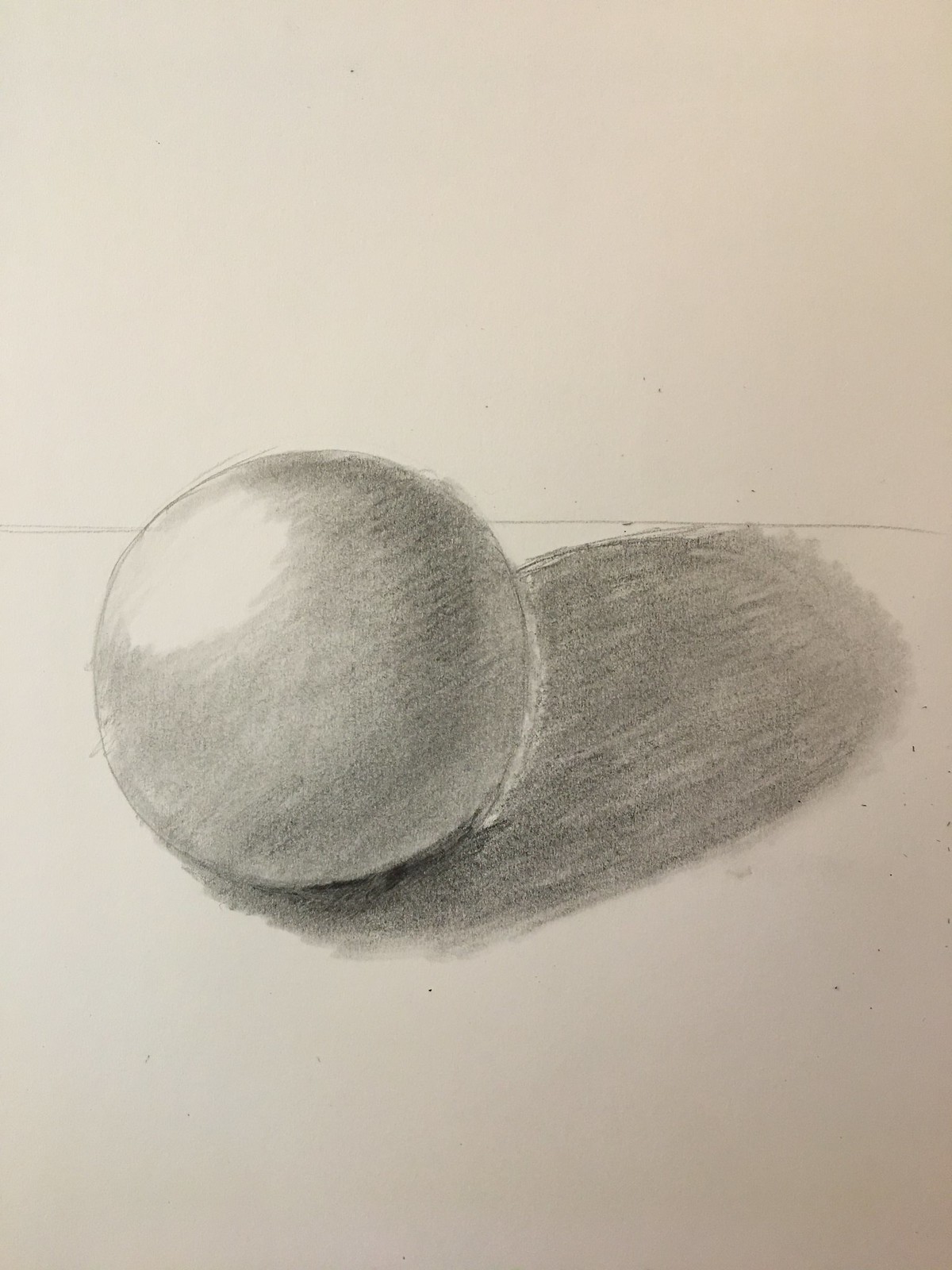The image depicts a detailed 3D sketch of a spherical object on a light gray piece of paper. The ball, primarily shaded in gray, features a gradient with the center darkened slightly with black tones. A striking beam of white light highlights the top left portion of the sphere, creating a realistic effect. The right side of the ball is thoroughly shaded, enhancing the illusion of depth. A horizontal line is subtly drawn across the top of the sphere, contributing to its dimensionality. To the right of the ball, there is an oval of shaded gray, resembling a shadow cast by the object. The background consists solely of the light gray paper, providing a stark contrast that emphasizes the intricate details of the sketch.